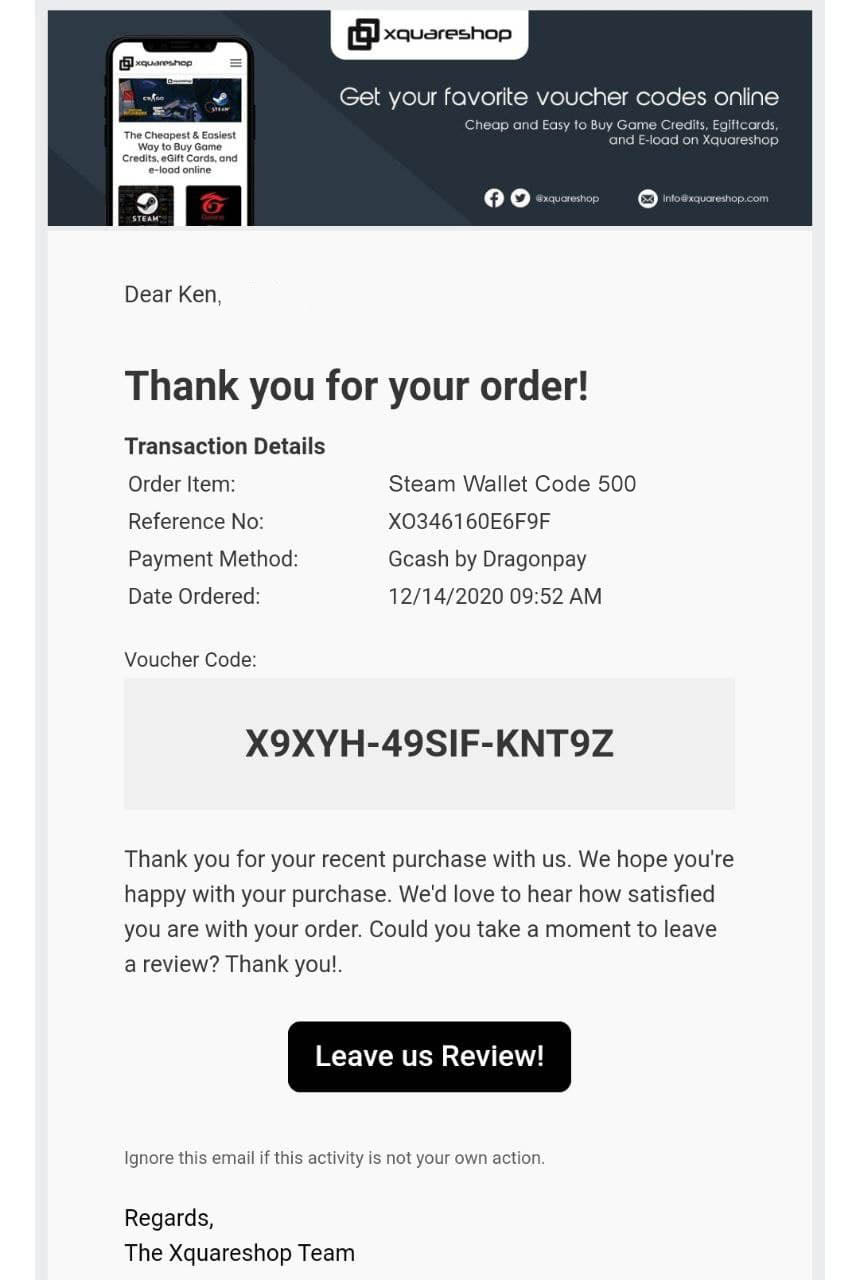This image is a detailed screenshot from a website called X Square Shop, prominently featuring its logo at the top center. On the left side of the screenshot, there is a digital illustration of a phone displaying the X Square Shop's tagline: "The cheapest and easiest way to buy game credits, e-gift cards, and e-load online." To the right, the website advertises: "Get your favorite voucher codes online, cheap and easy to buy game credits, e-gift cards, and e-load on X Square Shop."

Below this promotional content is an order confirmation addressed to a customer named Ken. The message thanks Ken for his order and provides detailed transaction information. The order item is a "Steam Wallet code 500," accompanied by a reference number and payment method, which is GCash by DragonPay. The order was placed on December 14, 2020, at 9:52 AM. Alongside this information is the voucher code necessary for using the Steam Wallet on the Steam platform.

The message continues with a note of gratitude for Ken's recent purchase and expresses a desire for customer feedback, inviting Ken to leave a review through a prominently displayed button labeled "Leave Us a Review". The email concludes with a caution to disregard the message if the activity was not undertaken by the recipient, signed off with best regards from the X Square Shop team.

The screenshot does not disclose the amount Ken paid for the Steam Wallet code.